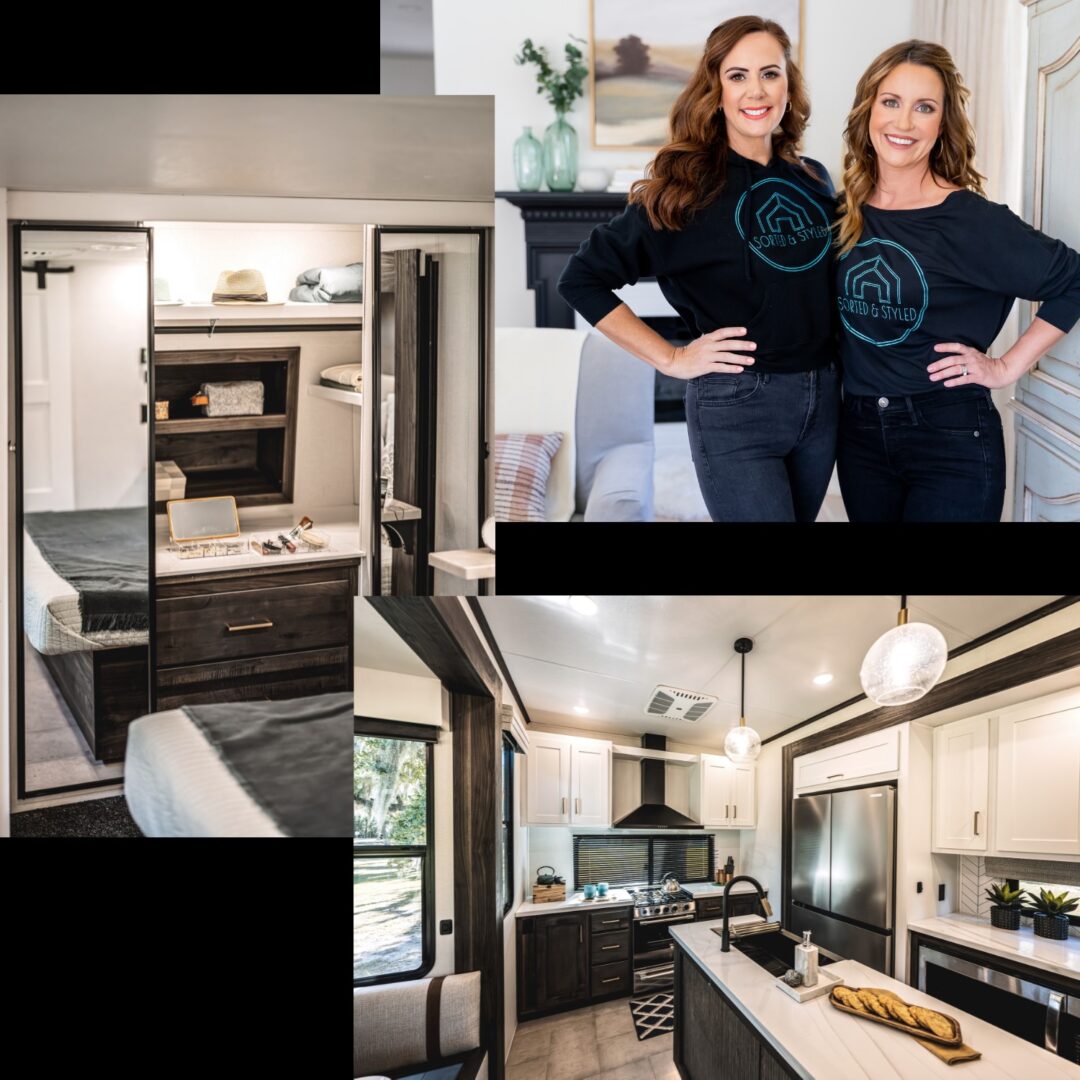The image is a real estate advertisement featuring a collage of three distinct photographs that highlight various parts of a home. At the top of the collage, there is a picture of two smiling, Caucasian women with brunette hair, both wearing identical sweaters that have a circular logo with the words "Sorted and Styled" and an image of a house. They are standing in a cozy, warmly-lit living room with a black-mantled fireplace adorned with flowers and a picture frame. The middle photograph showcases a bedroom with double mirrors where a bed and a vanity area are reflected. This room also features a small dresser, and the overall design maintains a stylish and cohesive decor. The bottom photograph captures a modern, rectangular kitchen with an island in the middle that has a sink and fresh-baked bread on it. The kitchen is equipped with a large double-door freezer fridge, a wine fridge, a stove along the back wall, and cupboards. The walls and ceiling are white, accented with black trim, and feature ceiling lights and a vent.